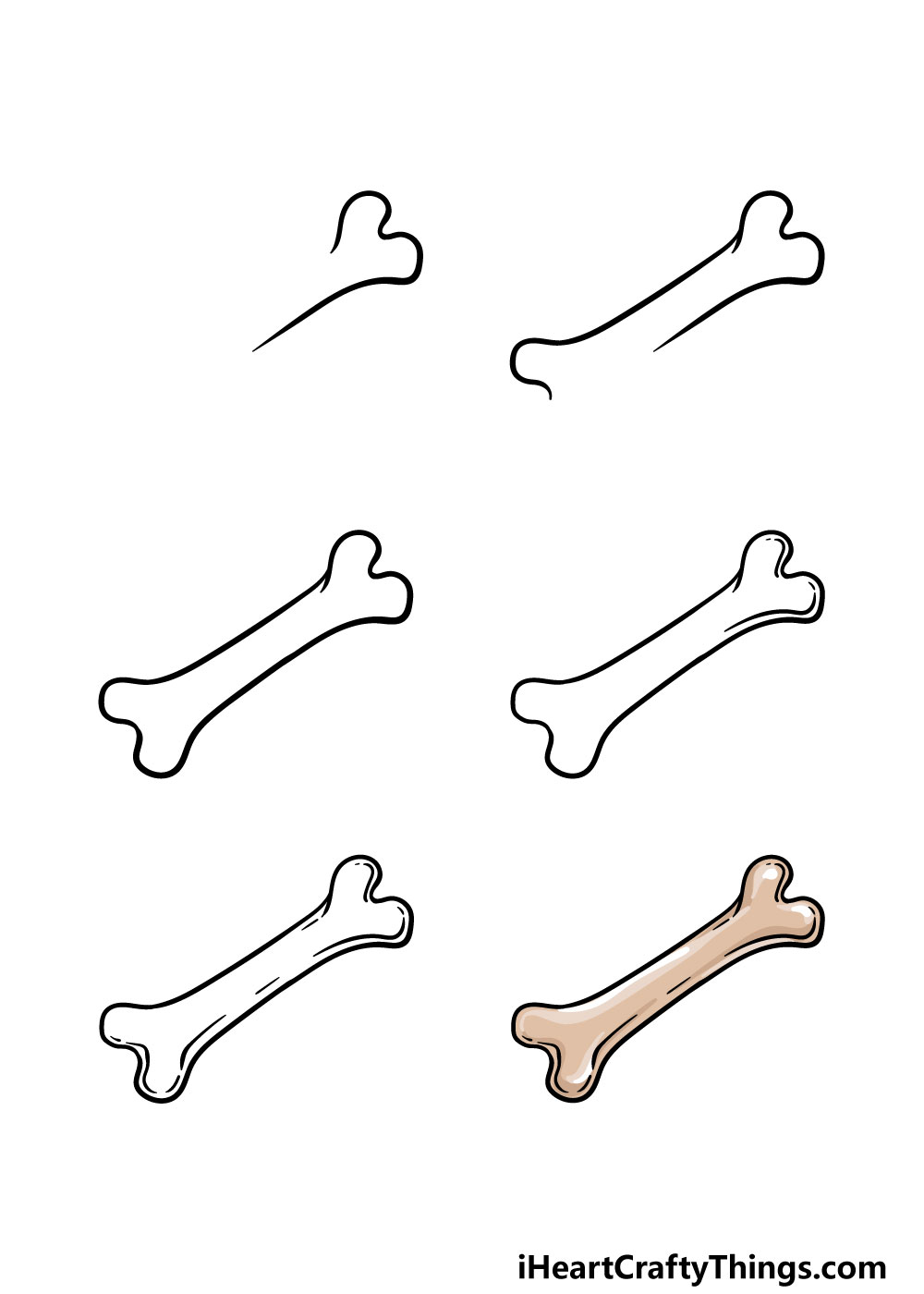This digital graphic image features six pencil-sketched dog bones arranged on a white background. These bones are lined up in two columns, with three bones in each column. Notably, the bone in the upper left corner is incomplete, missing one end. The bone in the lower right corner stands out as it is colored in brown, while all the other bones remain in pencil sketch form, with shades of white and grey. Below the colored bone is the text "IHeartCraftyThings.com," indicating the source website where this image can be found.